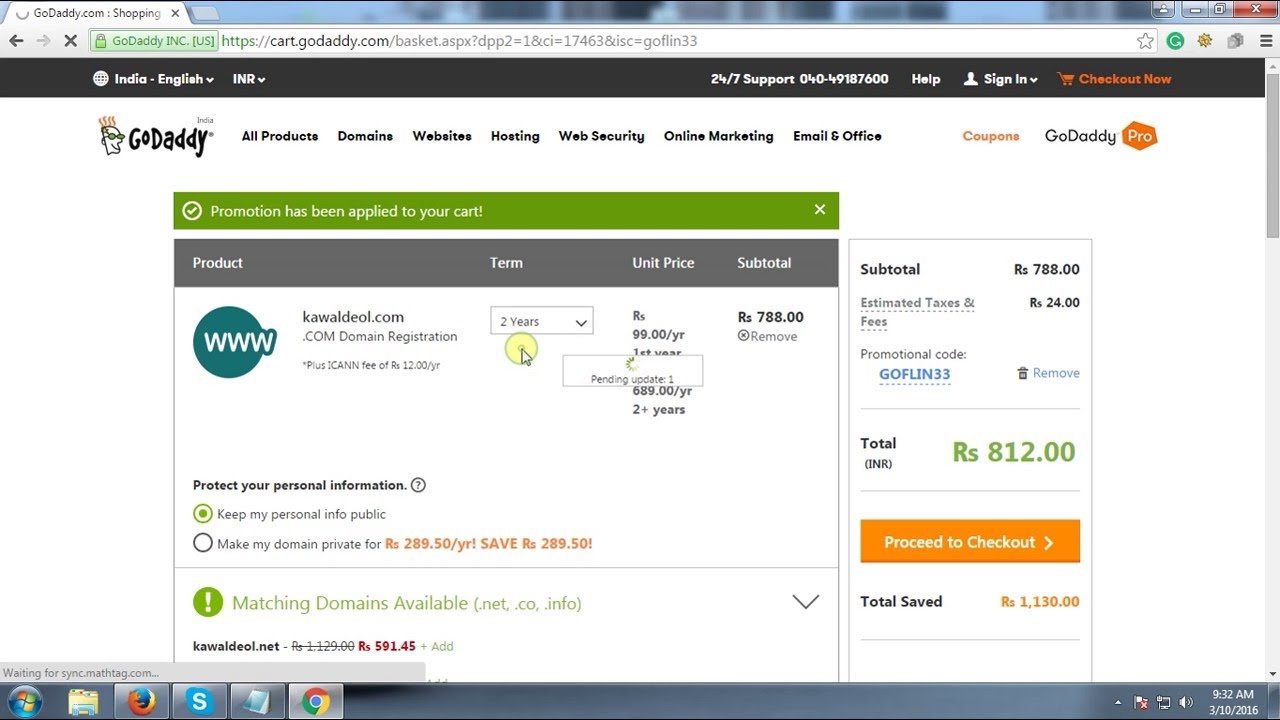A detailed screen capture from a computer monitor showcases a user purchasing a domain on the GoDaddy website. 

**Top Navigation:**
- **URL & Tab:** The browser tab reads “GoDaddy.com Shopping,” with the URL showing that the user is indeed on the GoDaddy website.
- **Header:** A black horizontal bar displays “India - English” and currency as "INR" with dropdown buttons for both. The top right corner features a phone number for 24/7 support, a “Help” option, a dropdown for “Sign In,” and a red “Checkout Now” button with a shopping cart icon.

**Main Section:**
- **GoDaddy Logo & Menu:** The upper left area features the iconic GoDaddy logo with a quirky character sporting glasses and distinctive hair. A navigation menu lists options for All Products, Domains, Websites Hosting, Web Security, Online Marketing, and Email & Office in black fonts. An orange "Coupons" link is presumably clickable, followed by "GoDaddy Pro" with a red hexagon icon.
- **Notification Bar:** Below the menu is a green-highlighted notification with a white checkmark, stating, "Permission has been applied to your cart."
- **Product Overview:** A gray banner underneath outlines the product details:
  - **Columns:** "Product" on the left, “Term” in the center, "Unit Price," and "Subtotal" on the far right.
  - **Purchase Details:** The user has bought a domain for two years costing ₹788.
  - **Privacy Options:** There’s a section about protecting personal information with a toggle option to either hide it for a fee or leave it public for free.
  - **Matching Domains:** A green circle with a white exclamation mark indicates matching domains available (.net, .co, .info), noting that KAWALDEO.NET has been registered.
  - **Subtotal & Discounts:** The approx. subtotal includes a domain (₹788), with the coupon code "GOFLIN33" applied. A trash can icon allows for removal.
  - **Final Amount:** The total cost is ₹812. Beneath, an orange “Proceed to Checkout” button stands out with yellow text. Below this, a note indicates that ₹1130 has been saved in total.

**Windows Taskbar:**
- **Icons:** The gray taskbar at the very bottom includes the Microsoft logo, File Explorer, Firefox, Skype, Notepad, and Chrome icons.

This image capture comprehensively details a domain purchase on the GoDaddy website, highlighting navigation elements, product details, privacy options, matching domain suggestions, and the final cost breakdown.